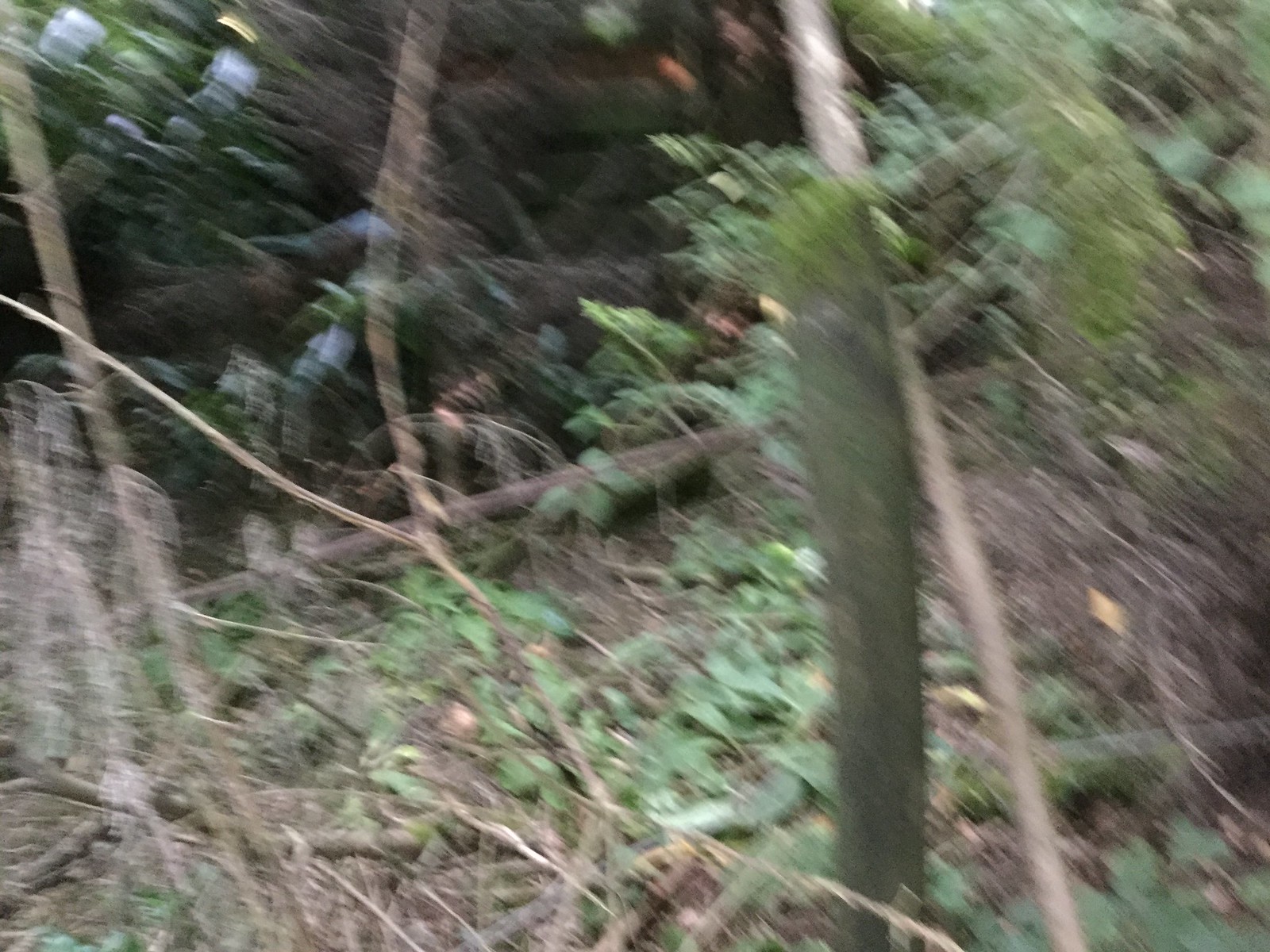An extremely blurry photograph of a nature scene, taken outdoors in what appears to be a wooded or overgrown area. The image captures the ground at a downward angle, making it difficult to assess the overall density of the forest. Scattered across the green grass are a mix of small, tan-colored downed branches. The ground also shows some weedleaf foliage. Slightly right of the center stands a larger, vertical tree stump with a grayish hue. In the upper right corner, blurry branches overhang from above, adding to the chaotic nature of the scene. The upper left quarter of the image is significantly darker and heavily shadowed, suggesting the presence of a denser area of foliage.